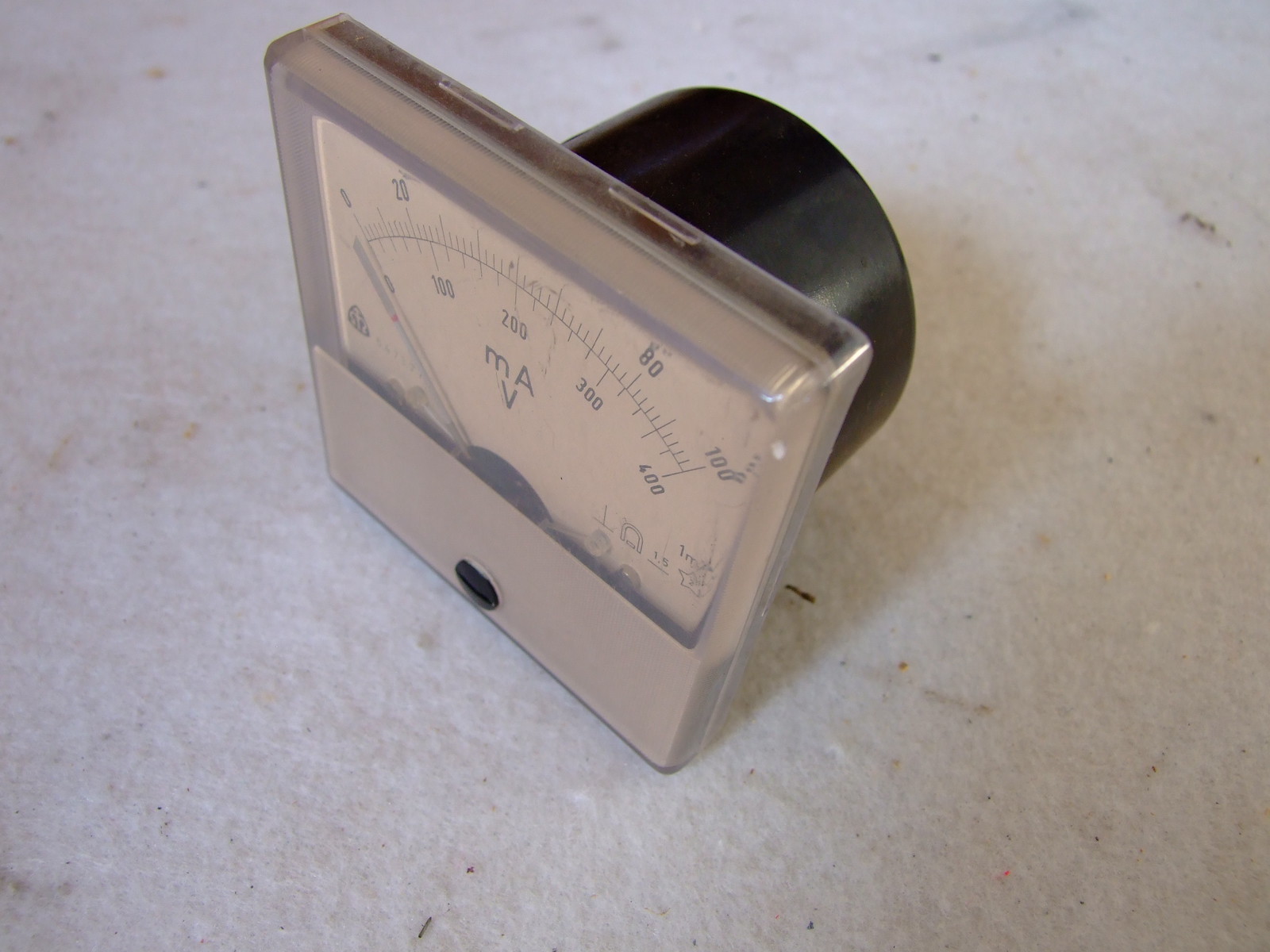This image features an aging gauge device positioned on a plain, speckled white floor. The gauge itself appears to be either a square or rectangular shape and is primarily gray. Prominently displayed at its center are the characters "mAV," with the 'm' and 'v' in lowercase and the 'A' in uppercase. The device has a small, circular black sensor at its lower section and is backed by a short black tube.

The gauge's top dial spans a numerical range from 0 to 100, with visible markers at 0, 20, 80, and 100. Below these, an extended scale ranges from 0 to 400, marked at 0, 100, 200, 300, and 400, with the 400 and 100 markers aligning precisely with the 0 and 20 markers on the top scale. Toward the bottom right of this scale, the number 1.5 is displayed, accompanied by a star and additional small symbols including an upside-down T and an inverted horseshoe. These symbols are positioned to the left of the 1.5, while the star is positioned to its right.

Above the 1.5 marking, there is another label reading "1M." The device shows signs of wear, including smudges on its plastic front, obscuring some text. Based on its appearance, the gauge seems to be a vintage piece, likely from the 1970s or 1980s, and it is currently disconnected from its original operational setup.